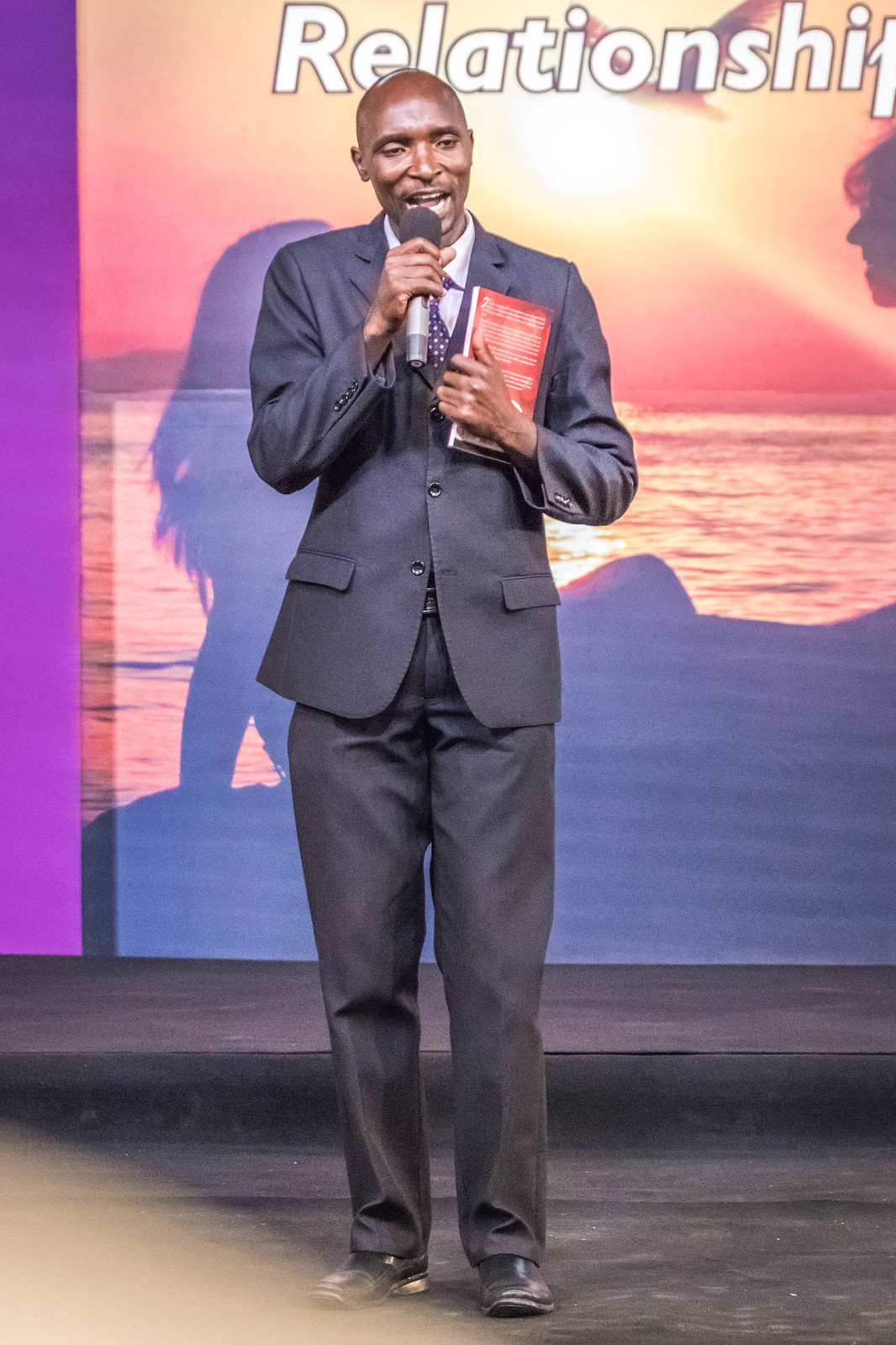In this photograph, an African American man, likely middle-aged and bald, is standing on a stage, dressed in a gray suit paired with a white shirt and a purplish polka-dotted tie. He looks incredibly professional as he addresses a crowd. His right hand holds a red book with white writing, though the title is obscured by his hand, while his left hand brings a microphone close to his mouth as he speaks.

The stage floor is black, and behind him is a wall with a projection screen. The screen shows a PowerPoint slide featuring the silhouettes of a woman and a man against a serene backdrop of water at sunset, with a bird flying in the sky. The background text is partially visible and prominently displays the word "Relationship." The poster and projection contribute to a soft ambiance with hues of purple, blue, and gold, suggesting a thematic focus on relationships.